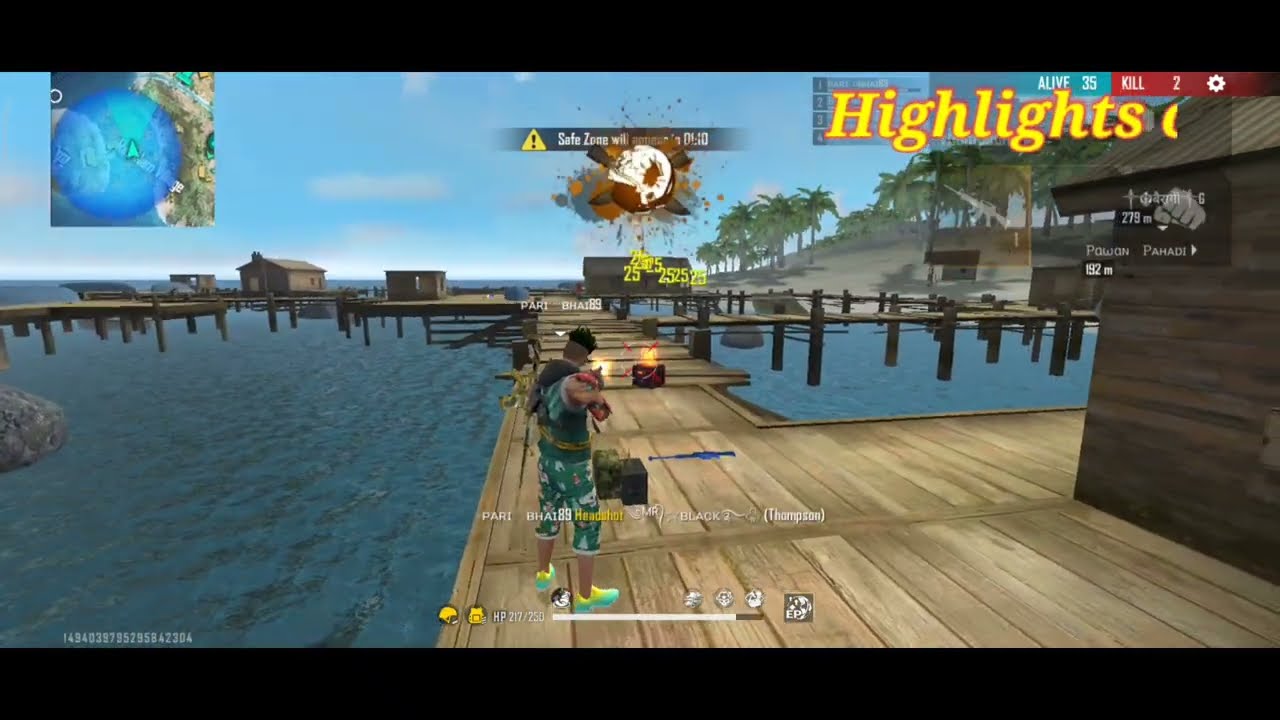This image is a screenshot from a third-person shooter video game, potentially Fortnite, showcasing a tropical island setting with numerous wooden piers extending over the water. The main character, a man depicted from behind, is aiming his gun at a brown box situated on the pier. He wears distinctive green Hawaiian-style shorts, a sleeveless green tank top, and green and yellow shoes. His head is shaved around the sides and back, with a curly mop top on top. The pier itself is made of light brown wood and has areas to dock boats on either side. In the foreground, you see status bars, progress bars, and a small map in the upper-left corner indicating the character's location. The background features buildings built on the water, a hill with palm trees, and a distant view of a blue sky dotted with white clouds. Explosions and animated effects are visible in the distance, adding to the dynamic scene. In the upper-right corner, the text "highlights" is displayed in yellow, along with "live 35 kill 2," suggesting an ongoing game session with specific stats.